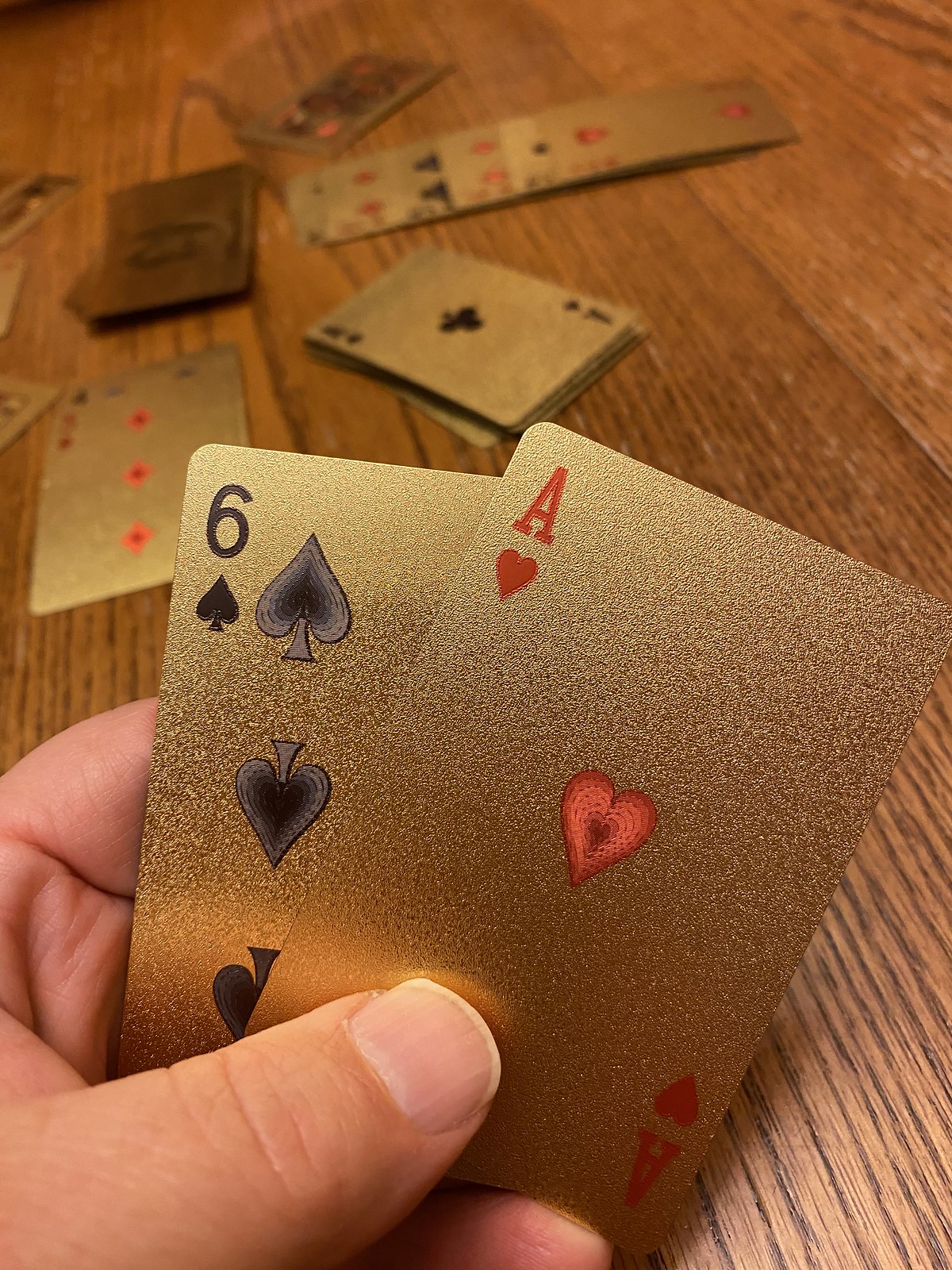In this cozy setting inside a home, a card game is unfolding on a classic wooden table. The focus is on a person's hand, holding up two distinctive golden cards towards the camera: an Ace of Hearts and a Six of Spades. In the background, various stacks of cards blur, giving a sense of depth and activity in the game. Among these piles, one prominently displays an Ace of Spades and a Three of Diamonds, with a visible pattern alternating between black and red suits. The intricate details of the game remain a mystery, but the scene captures the essence of a leisurely and engaging moment shared over an intriguing card game.